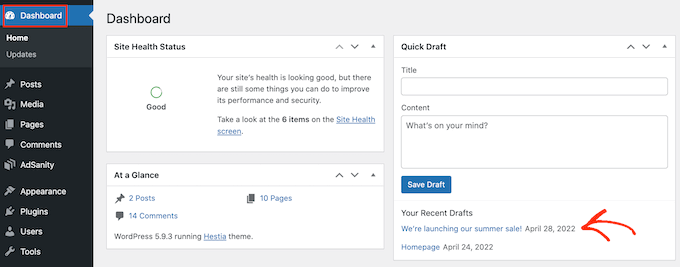This image is a screenshot of an administrative interface of a website's backend dashboard. The top section of the screen displays a toolbar, alongside a vertical sidebar on the left. The sidebar, styled with a black background and white text, lists various menu items including: "Dashboard," "Home," "Updates," "Posts," "Media," "Pages," "Comments," "Add Sanity," "Appearance," "Plugins," "Users," and "Tools," each accompanied by distinct icons.

Centrally, beneath the "Dashboard" header, the "Site Health Status" is prominently displayed, indicating a "Good" status, visually reinforced by a green ring encircling the word "Good." Below this status, a paragraph advises that, although the site's health is favorable, there are opportunities to enhance performance and security. It directs the user to review six specific items on the Site Health screen, with "Site Health screen" presented as a clickable link for further action.